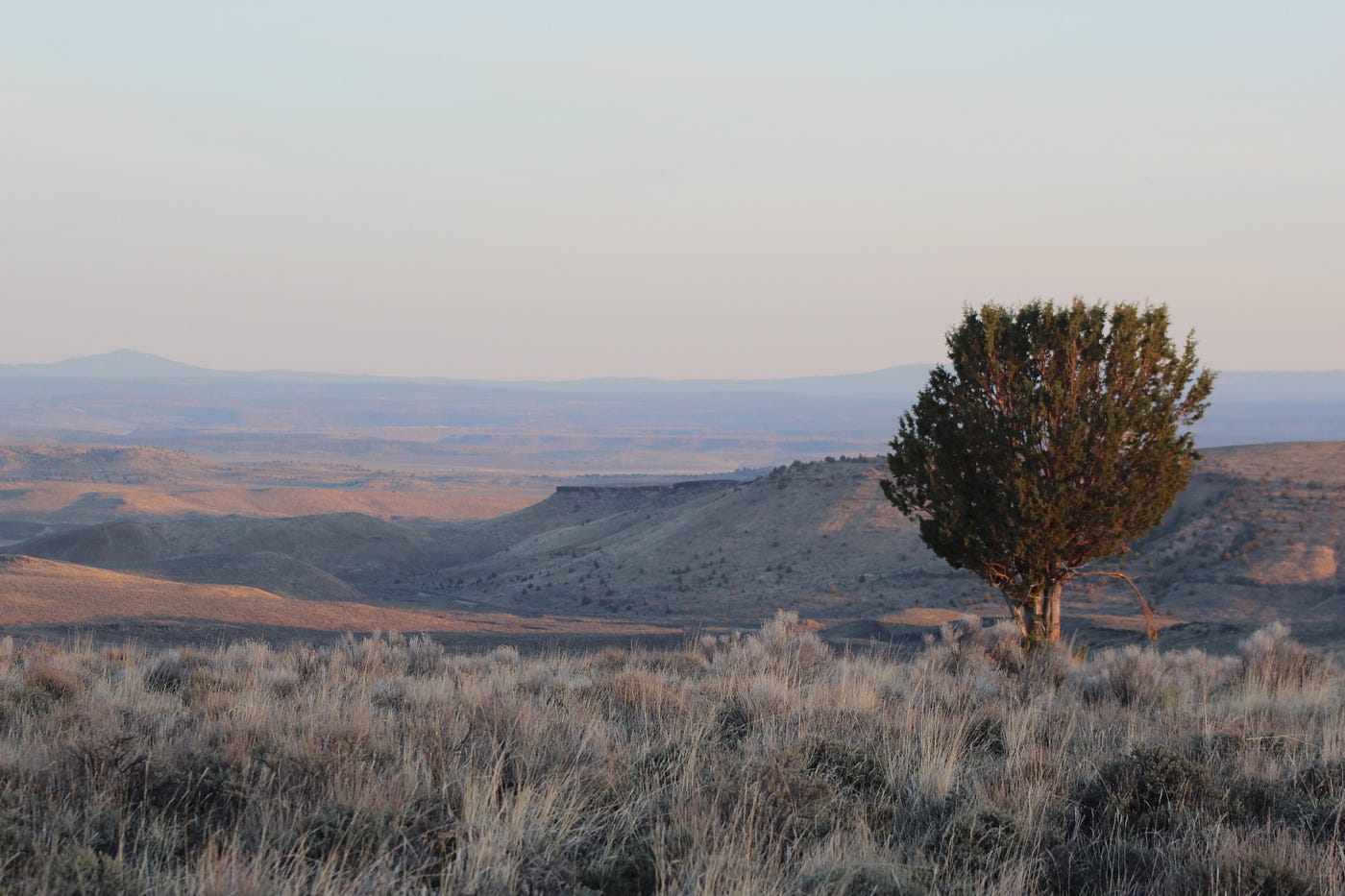This landscape-oriented photograph captures a serene and expansive terrain that harks to the western United States, potentially resembling areas like Joshua Tree or regions in Nevada or Arizona. The scene is framed by a gentle descent over a grassy hill adorned with tall, grayish-brown grass suggestive of late spring or early fall. On the right-hand side stands a fir tree, whose mostly green leaves are tinged with brown, hinting at seasonal transition. The foreground stretches into a valley, transitioning to rolling hills dotted with additional greenery, eventually leading up to a mountainous backdrop.

The lighting in the image is soft and diffused, with a subtle haziness that envelops the horizon, enhancing the late or early day ambiance with light blue and pink hues. Shadows cast by the sun suggest it is positioned to the right. In the more central background, ambiguous shapes—which may be either animals grazing or distant structures—add an element of intrigue against the vast, open space. The tallest mountain stands prominently on the left, with a series of smaller mountains trailing to the right, all bathed in the golden light of an early evening or a similar tranquil time of day, further contributing to the timeless and expansive feel of the landscape.